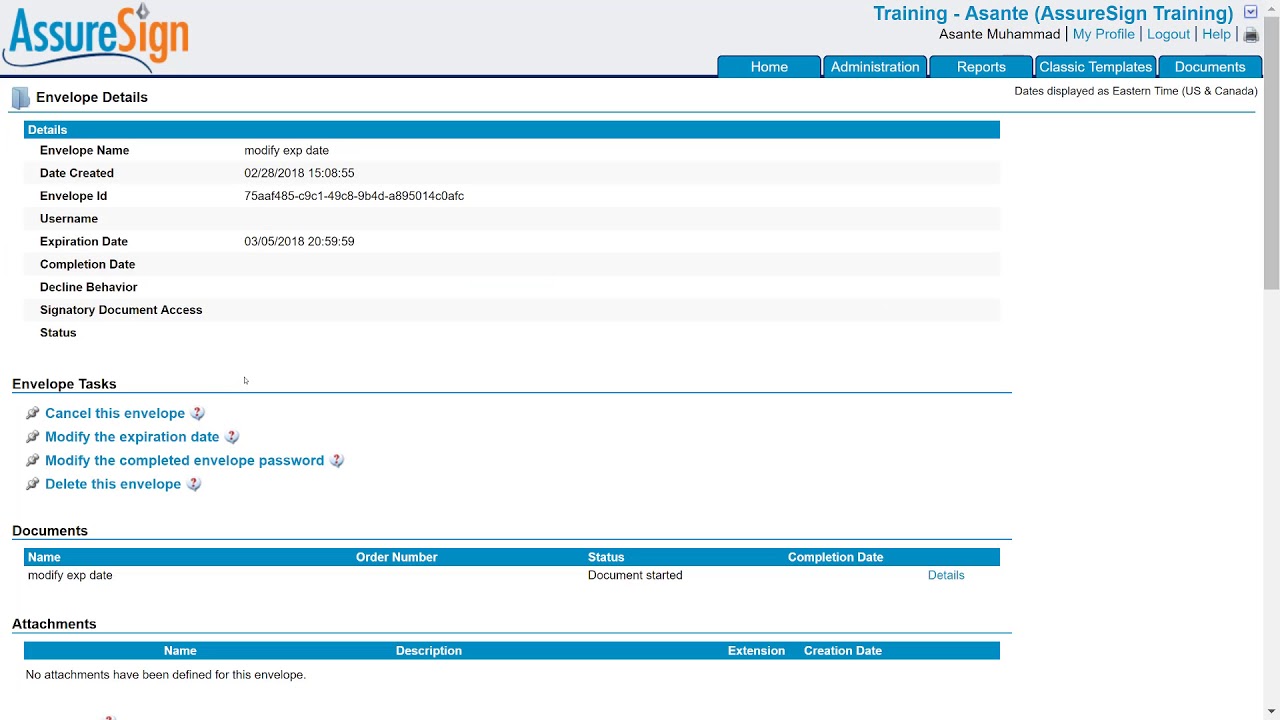This cropped screenshot captures a detailed view of the AssureSign desktop app's training page. At the top of the page, a gray header prominently features the AssureSign logo on the left. On the right side of the header, the username "Training Asante" is displayed with "AssureSign Training" in parentheses beside it. Directly below this, on the center right, the username appears once more, accompanied by blue navigation options: "My Profile," "Logout," and "Help."

The interface's main navigation bar, situated beneath the header, is characterized by five blue tabs: Home, Administration, Reports, Classic Templates, and Documents. The primary body of the page is white, showcasing four distinct categories.

On the far right of the screenshot, a thick gray scrollbar reveals that the page is currently scrolled to the top, indicating additional information can be accessed by scrolling down. 

At the top left of the page, the section titled "Envelope Details" is marked by a blue bar labeled "Details," which precedes a vertical list of detail entries. The next section, "Envelope Tasks," features a vertical list of tasks set against a light blue background. The categories "Documents" and "Attachments" follow, with the latter visible at the bottom of the screenshot, both currently displaying no listed items.